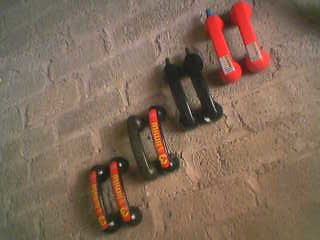This photograph, captured in color, displays four pairs of objects resembling hand weights, arranged on a concrete floor presented with a brick-like pattern marked by light gray grout lines. The slightly weathered surface shows cracks in the grout, providing a rugged backdrop for the array of weights. The objects, which double as ergonomic hand handles for push-ups, ensure added support and prevention of slippage during exercise. The topmost pair is fluorescent orange with white tags on the ends. Below them, a black pair sits unadorned, followed by another black pair featuring a red rectangle with yellow writing and a digit '3.' The bottom pair is also black, sharing the same red and yellow label, creating a uniform but strikingly structured alignment over the rugged concrete floor.